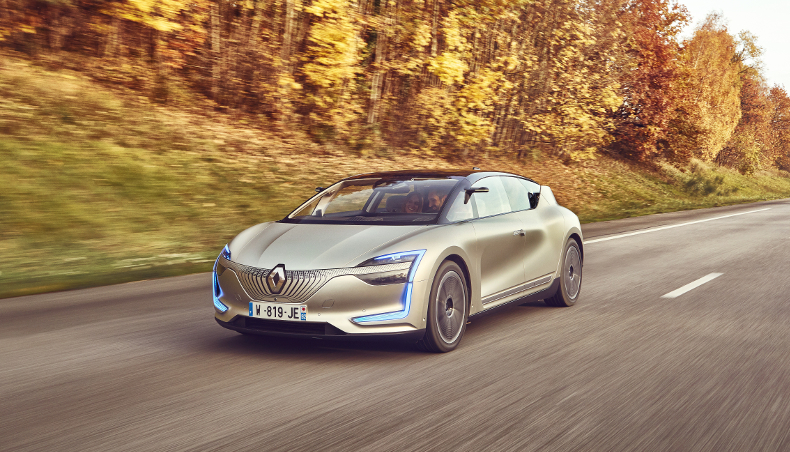The photograph features a silver Renault car driving towards the viewer from the center right, heading down toward the bottom left corner of the image. The car has a distinctly modern and sleek design, with a low stance and a windshield set at a sharp angle. Its silver exterior is complemented by blue accents around the headlights and intricate silver rims that appear blurred due to the car's motion.

In front of the car is a white license plate bearing the numbers and letters "W819 JE," revealing its European origins. Inside the car, there are two passengers: a male driver and a female companion seated to his left. The car's out-of-focus background suggests it is speeding along an asphalt road lined with tall trees blanketed in yellow and orange autumn leaves. The trees, situated on a grassy slope to the left of the road, add to the dynamic, picturesque scenery as the car travels through this vibrant landscape.